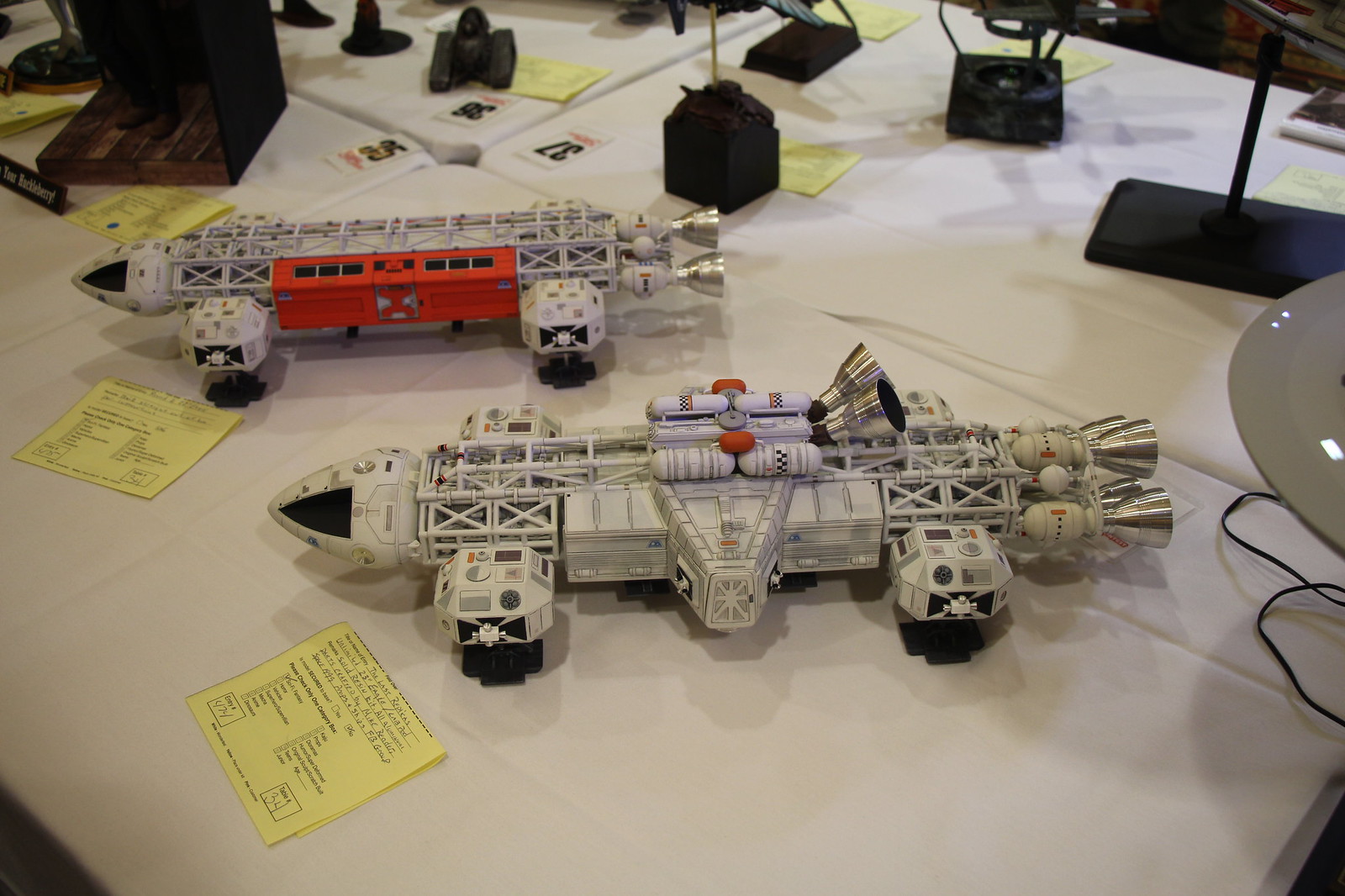The image features two detailed Lego Star Wars spacecraft models placed on a large white tablecloth that spans across four tables put together. Each model boasts unique colors and intricate components: one is primarily off-white with subtle gray and orange details, while the other has distinctive red markings on its side. Both models are elevated on black stands and equipped with thrusters, with a seeming focus on detailed design elements such as cockpits, boosters, and side pods that could serve as living quarters or emergency shuttles.

The table is dotted with numerous yellow labels featuring handwritten notes, marking the items as part of a display or competition. These labels are positioned in front of each spacecraft and among the black, tall pieces scattered across the table, indicating a level of organization. Numbered place cards (35, 36, and 37) are also visible, further suggesting an event setting, possibly a science fair. Additionally, a lamp with a visible cord is placed to the side, casting light on the detailed models. The overall scene is set indoors, with the photo taken at an angle to capture the entirety of the display.